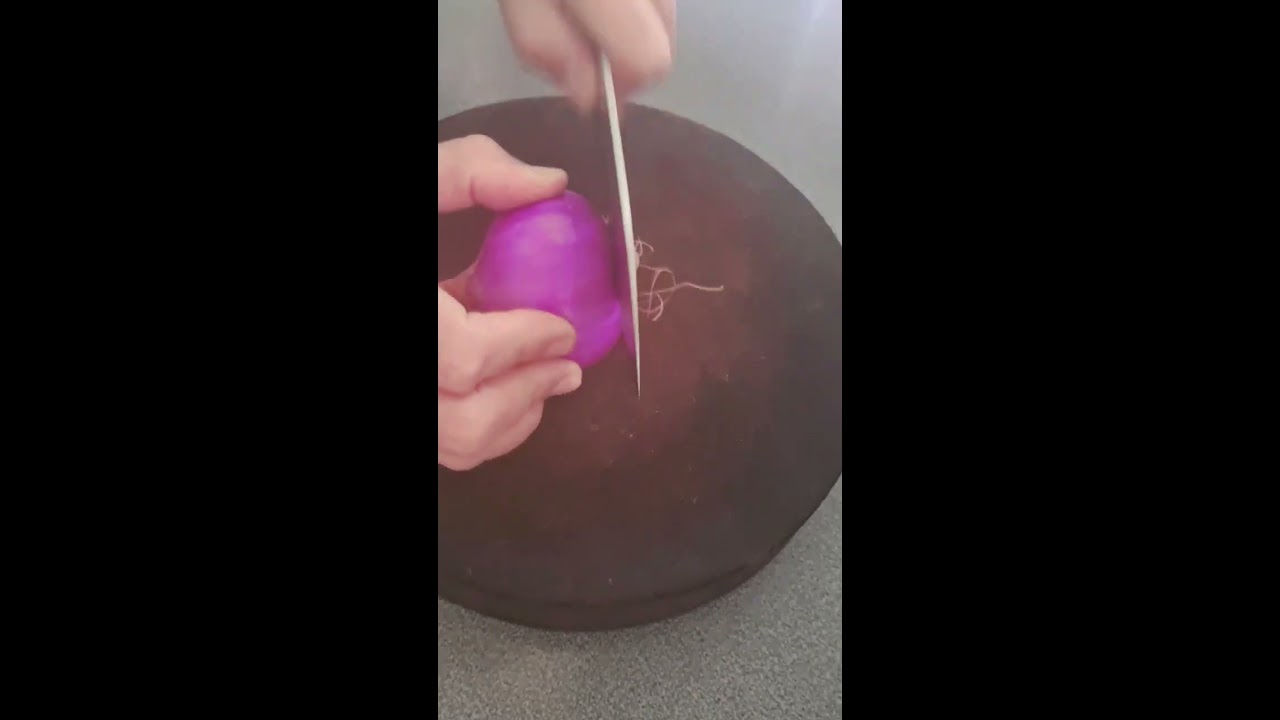In the image, we see an outdoor scene during the daytime, focused on a person's hands as they prepare to cut a red onion, which is visually purple in color. The person's right hand grips the onion on its side, with their thumb on top and fingers around it, while their left hand holds a sizable knife, halfway through making the initial cut to remove the end with stringy roots. The cutting is taking place on a thick, round, dark brown cutting board, resembling a tree stump or butcher block, placed on what appears to be a gray, granite-like countertop. The rectangular image is oriented in a way that suggests it could be part of a cooking video, possibly for a platform like TikTok, and is flanked by thick black bars on the sides. This setup, combined with the mundane yet intimate detail of the preparation process, evokes the instructional feel of a recipe or cooking tutorial.